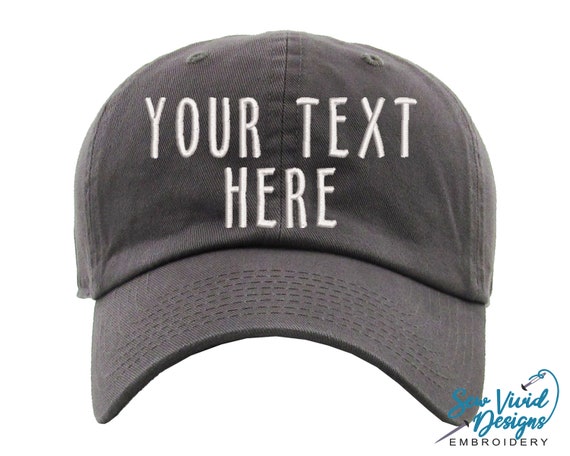This professionally shot close-up photograph features a dark gray, fabric snapback cap with a slightly curved brim. The cap prominently displays the customizable embroidered text "YOUR TEXT HERE" in white, all-caps font on the front. There is a vertical stitching line that splits the cap in half, and along the where the hat goes over the forehead, you can see eight horizontal rows of detailed stitching. On the bottom right corner of the image, the logo "SO VIVID DESIGNS" is elegantly written in cursive dark blue font, and below it, the word "EMBROIDERY" appears in small, black, all-caps regular font. Notable stitching and textural details enhance the visibleness of the fabric and craftsmanship of the cap. The image's blank white background emphasizes the hat as the central focal point.